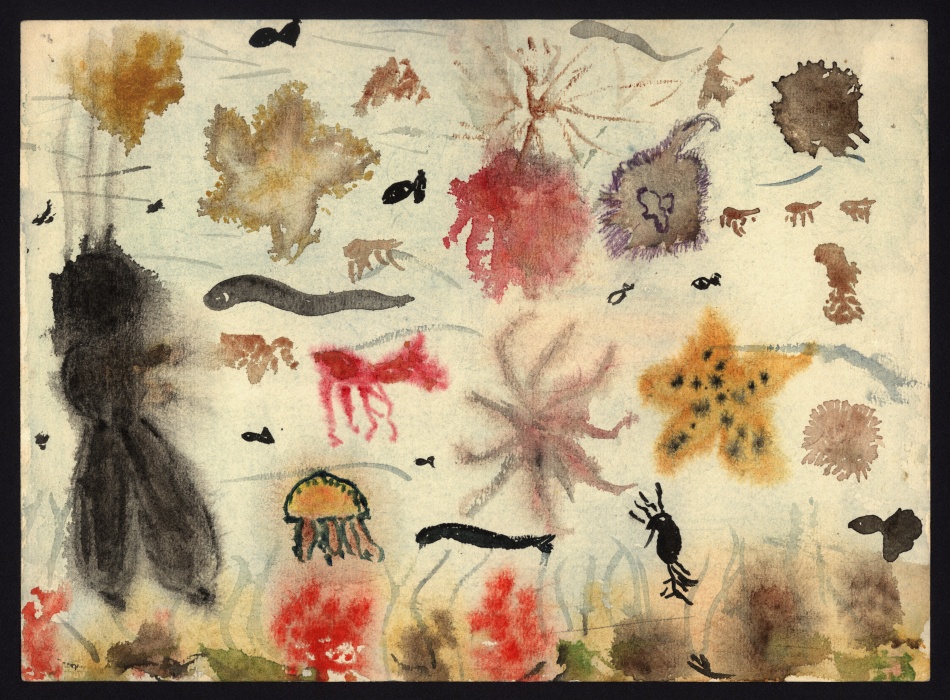The painting, framed with a black border, is done on beige, light brown-colored paper using watercolors and ink. This abstract piece features a colorful array of underwater and terrestrial elements. Dominating the scene is a yellow starfish dotted with black spots, and a yellow jellyfish adorned with black marks. There's an array of splotchy, somewhat indistinguishable sea creatures including sea anemones, a snail, worms, and some identifiable fish, all contributing to the chaotic underwater theme. The painting also incorporates an outline of a black moth, a snake, and hints of leaves or tree-like shapes, adding a fantastical element. The use of colors such as orangey-yellow, gray, red, green, and brown, particularly near the bottom, suggests coral or sea plants. The ink sketchings add sharpness to certain elements, juxtaposed against the soft, splotchy watercolor effects.